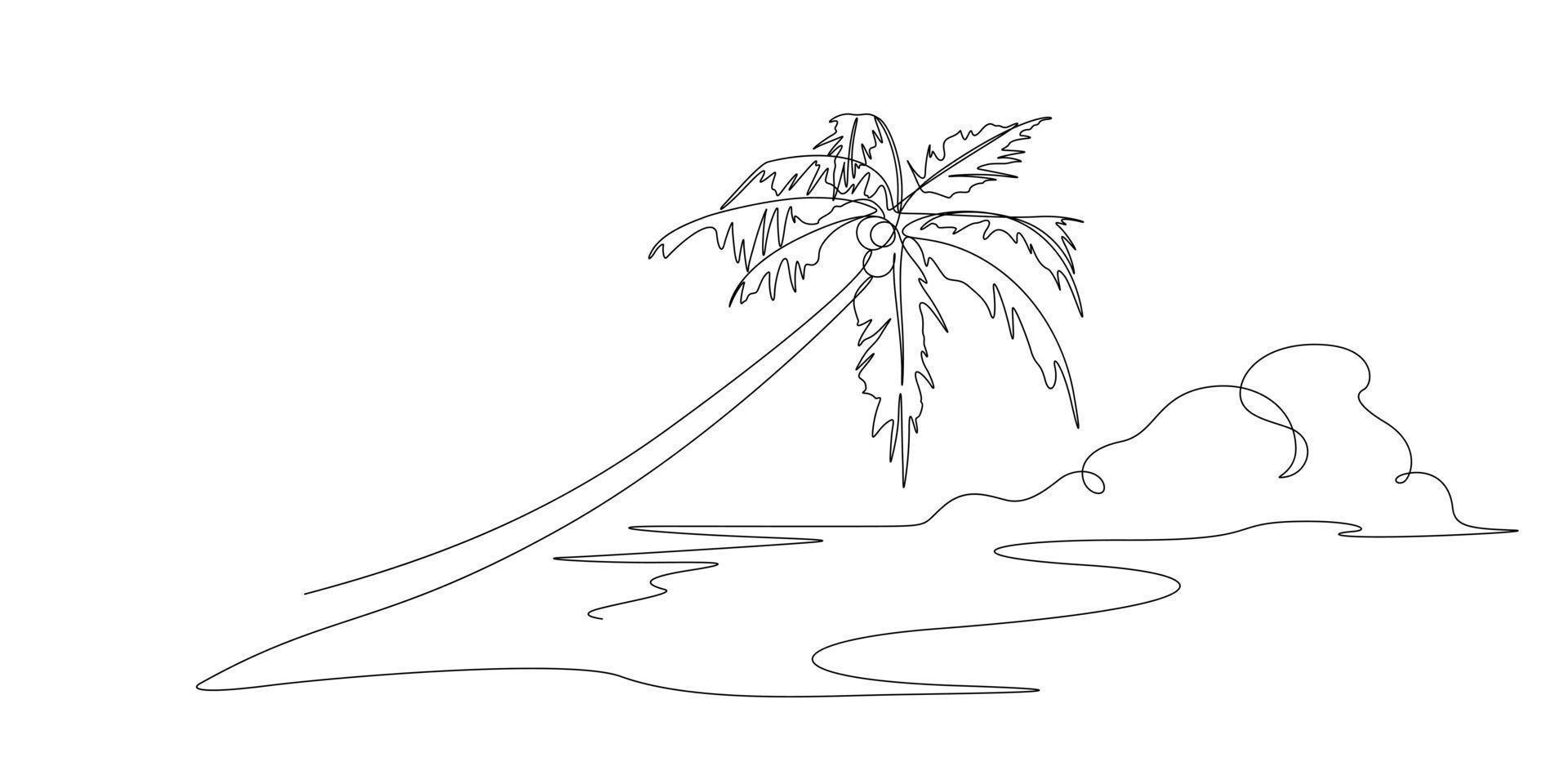This is a minimalistic, black-and-white line drawing on a bright white background, created with a single, continuous thin black line. From the bottom left of the image, the line forms an eight-leaved palm tree leaning diagonally to the upper right, with two coconuts nestled on its trunk. The palm leaves have a jagged edge, adding texture to the otherwise simplistic artwork. The line then continues downward and rightward, morphing into a series of loose, squiggly lines depicting a cloud. This cloud shape transitions into a sharper, zigzag pattern representing water towards the center of the page. The uninterrupted, flowing line seamlessly ties together the palm tree, cloud, and water elements in a cohesive, elegant design.